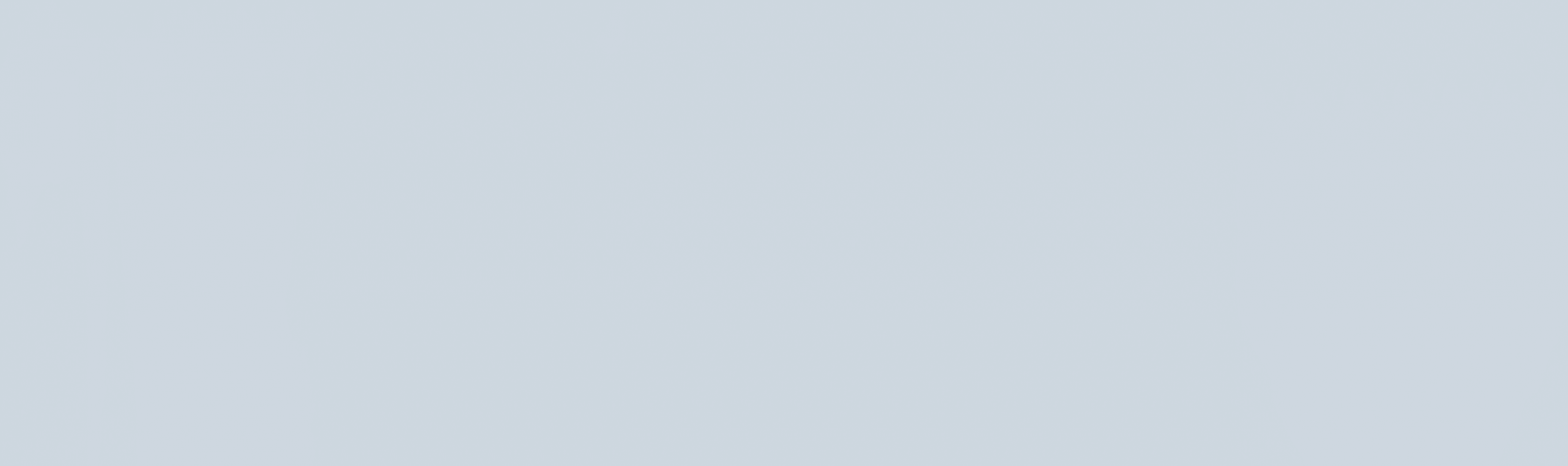The image depicts a screenshot featuring an entirely gray background devoid of any text, icons, or visual elements. While at first glance, it might seem simple and uninformative, this blank gray screen can carry significant implications, especially within the realm of Apple devices. In the context of Apple hardware, a gray screen is often referred to as the "dreaded gray background." This can be an ominous sign; without a progress bar, it might indicate a serious issue such as a failed hard drive or a malfunction within the motherboard. It could also suggest that the computer has encountered a hang-up due to overheating, aging components, or loss of thermal paste. However, in the given screenshot, it is hoped that the gray background is merely the default color in the image and not indicative of any underlying technical issue. The simplistic nature of the screen belies the complex array of potential concerns it could represent in a functional context.